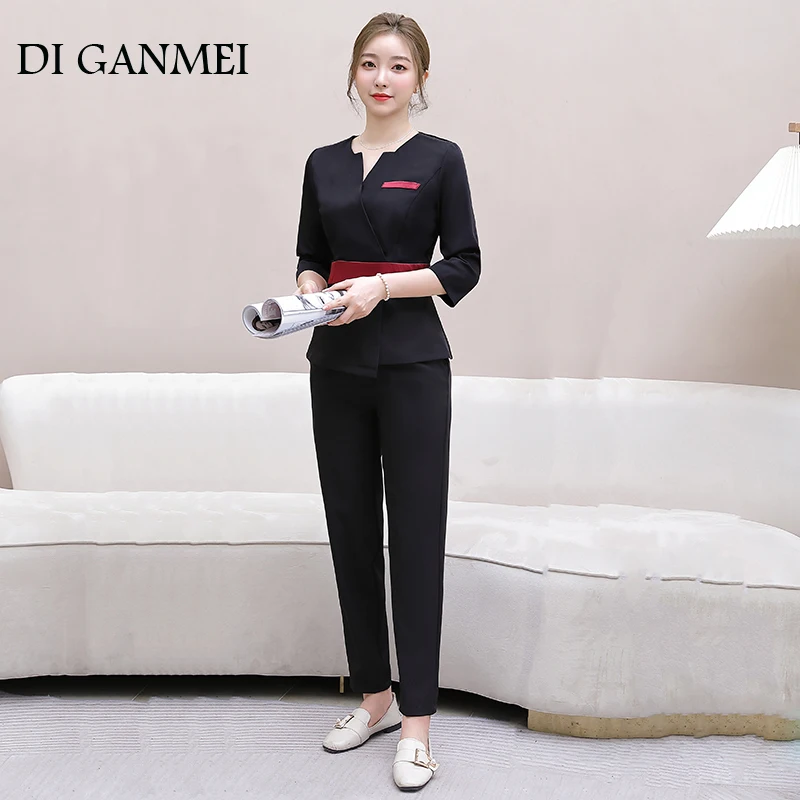The photograph showcases a young Asian woman with light brown, slightly pulled-back hair adorned with a few tendrils around her face. She's wearing red lipstick and exudes a demure smile. Her outfit consists of a black two-piece ensemble; the tunic top, featuring a V-neck and three-quarter length sleeves, is cinched with a red belt and accented with a red strip above the left breast pocket. Her pants are long and narrow, matching the black top. She complements her attire with cream-colored loafer shoes that have a gold band, a pearl bracelet on her left wrist, and white earrings. In her hands, she holds a rolled-up magazine.

The setting appears to be indoors, with the woman standing in front of a modern, cream-colored sectional sofa on a textured carpet. The background wall is a light tan, adding to the warm, neutral palette of the scene. A partial view of a pleated lampshade is visible on the right side. The image bears the text "D.I. GANMEI" in the upper left corner, suggesting it might be related to a fashion brand or campaign. Notably, there are signs of evident and poorly executed retouching on the right side of the sofa, creating a visible distraction in an otherwise composed scene.